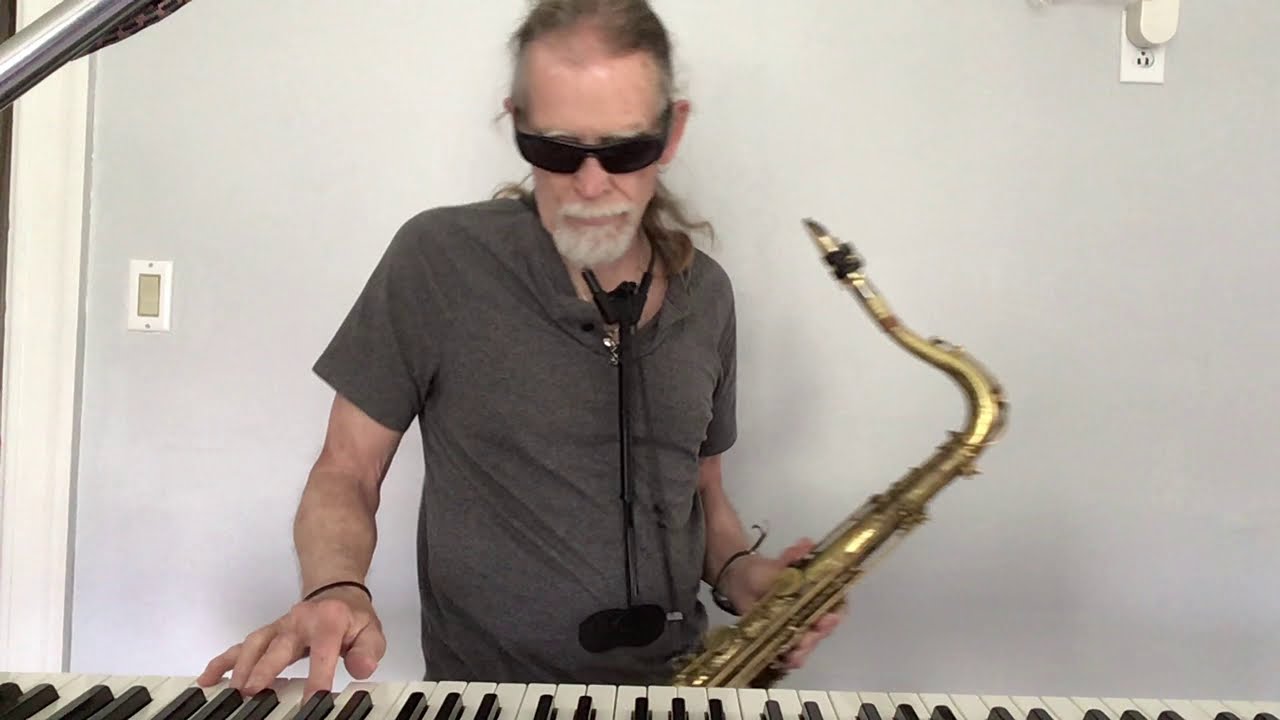The image depicts an older man, likely in his 50s or 60s, standing in the center. He has light brown to gray hair tied into a ponytail and sports a white or gray peppered goatee with a small beard. His eyes are hidden behind sunglasses. The man is dressed in a medium to dark gray short-sleeve t-shirt and wears leather bracelets on both wrists. In his right hand (viewer’s perspective), he holds a brass instrument, likely a saxophone, and his left hand is placed on the keys of a keyboard, which is situated in front of him. Not all the keys are visible, but many, particularly on the left side, can be seen. There's a black microphone around his neck. The background shows a pale bluish or lilac-colored wall, and additional details include a light switch and a power outlet, suggesting the setting is possibly a private music studio. The colors in the image are white, gray, black, tan, gold, and silver. The photograph is in landscape orientation, capturing the man from the waist up, and the overall style is representational realism.